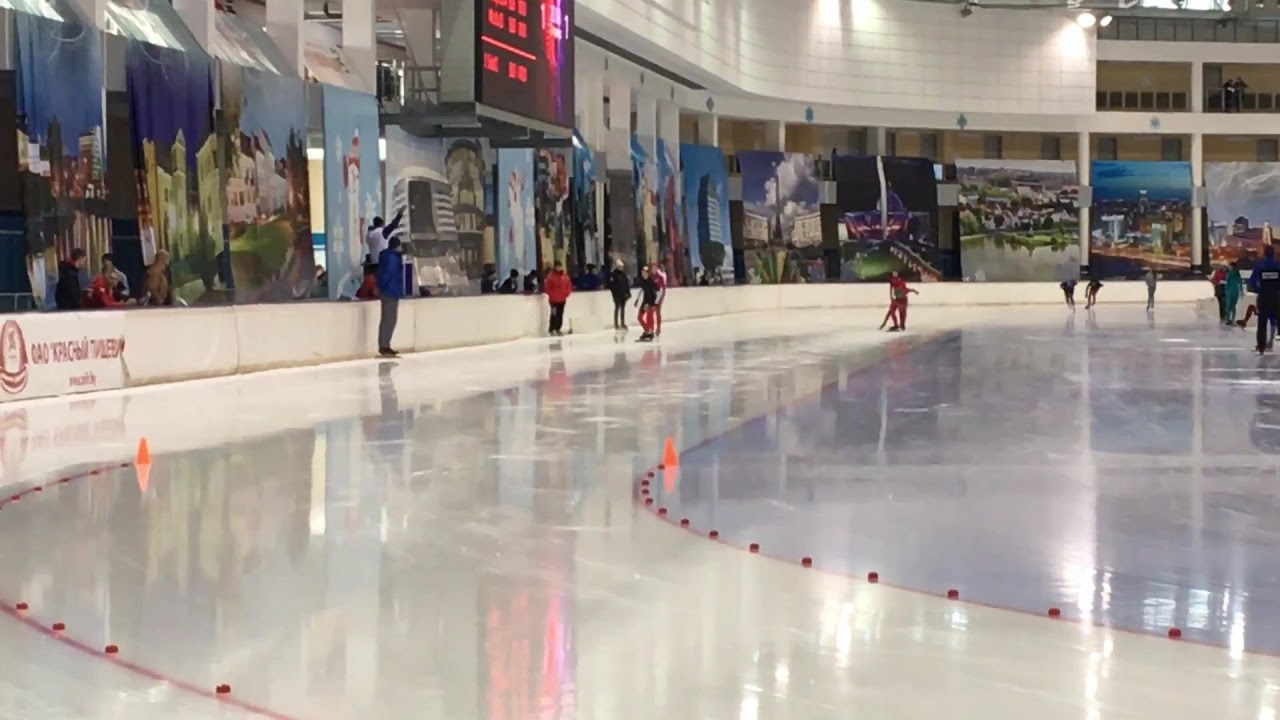The image captures a lively scene at an ice hockey rink. The ice rink's surface is pristine white and highly reflective, accentuated by red curved lines and dots that demarcate the various areas. Two small orange traffic cones sit on one side of the rink. Several players are on the ice: two in red jerseys who appear to be leading an ice skating race, and others wearing different colors including one in black. One player in a red jersey is notably holding a red badge. Surrounding the rink, the walls are adorned with numerous paintings and large banners. Above this, a black digital scoreboard with red scores prominently displays in the top center of the image, though the specific details on it are unreadable. The scene is vibrant, featuring an array of colors including blue, green, and purple amidst the dominant reds and whites.